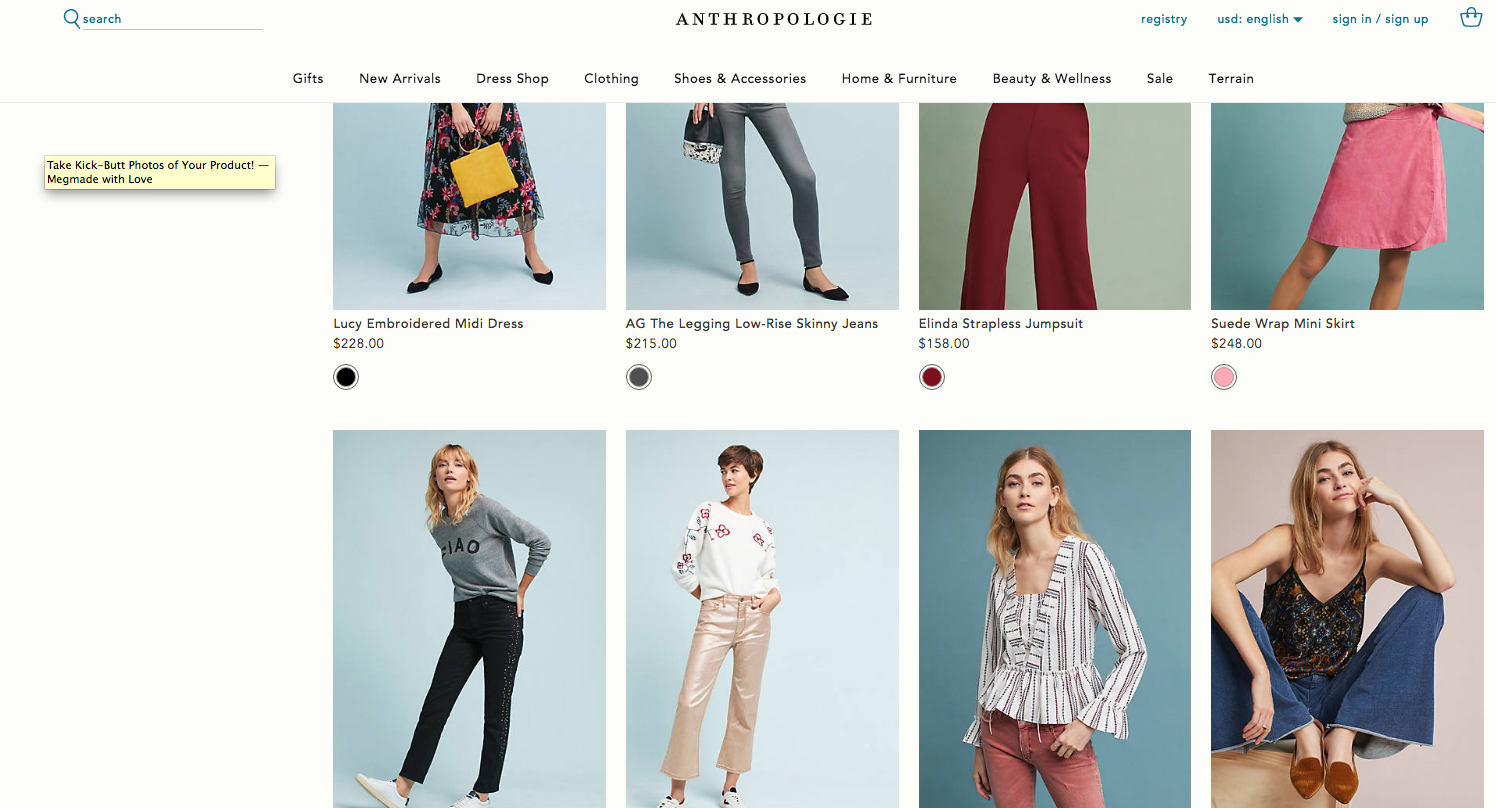Screenshot of an Anthropologie shopping webpage. The image features a clean layout with predominantly black text on a white background. In the upper-left corner, there is a search bar, and directly beneath it, a yellow box with black writing and a right-pointing arrow, seemingly superimposed on the page.

In the upper-right corner, options for registry, USD currency, English language, sign in, and sign up are visible. Below these options, a navigation bar lists categories: gifts, new arrivals, dresses, shop, clothing, shoes and accessories, home and furniture, beauty and wellness, sale, and Terrain.

The main content area displays eight product images, though only the bottom halves of the top four are visible. The products include:

1. A Lucien Brodert Midi Dress, priced at $228, depicted in black with pink flowers, paired with a square yellow handbag.
2. AG Leggings Low-Rise Skinny Jeans, priced at $215, shown in grey.
3. A Linda Strapless Jumpsuit in maroon, priced at $158.
4. A Suede Wrap Mini Skirt in pink, priced at $248.
5. A woman in a grey long-sleeved t-shirt and black skinny jeans.
6. Another woman in a white top with red flower detailing on the sleeves and beige leather trousers.
7. A woman with long blonde hair wearing a striped shirt with flared sleeves and red jeans.
8. A woman with long blonde hair wearing a strapless navy top with a floral print and wide-legged jeans or an ankle-length denim skirt, accompanied by suede brown pointed pumps.

All the women in the images appear to be Caucasian.